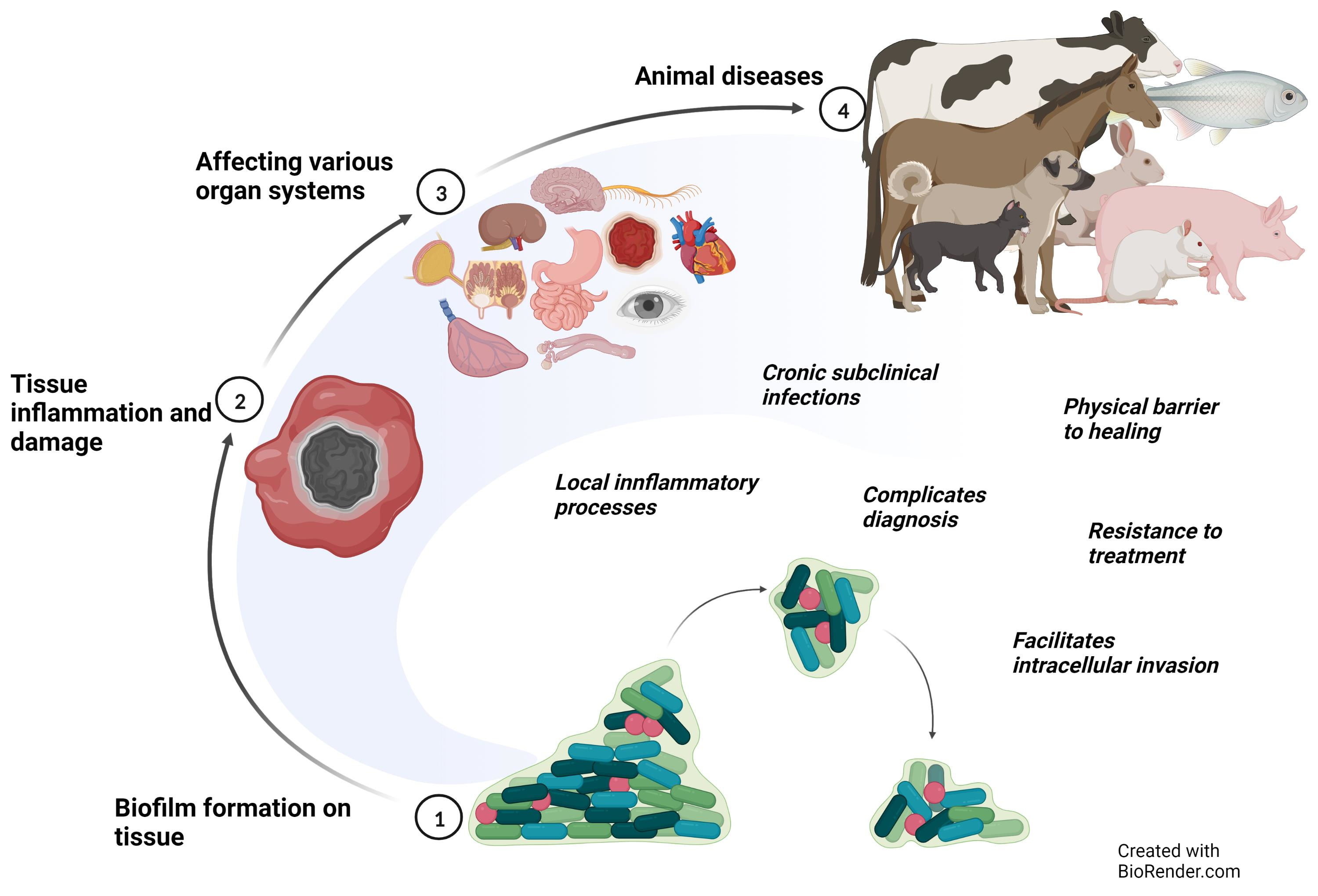The infographic, created with BioRender.com, provides a detailed visualization of the progression of a disease in animals through four distinct stages. Starting at the bottom center, Step 1, labeled "Biofilm formation on tissue," is depicted with blue, green, and dark green rods along with red circles, with an arrow movement from larger to smaller clusters. Step 2, found on the left, is labeled "Tissue inflammation and damage" and features a black spherical mass with a red exterior shell. Moving upward and towards the center, Step 3, "Affecting various organ systems," illustrates various organs in full color, including brains, livers, stomachs, hearts, and eyes. The final stage, Step 4, located at the top right, is labeled "Animal disease" and showcases a variety of animals, such as cows, horses, dogs, cats, pigs, rats, bunnies, and fish. Additional text dispersed throughout the image highlights complications including local inflammatory processes, chronic subclinical infections, complicated diagnosis, physical barriers to healing, resistance to treatment, and facilitating intracellular invasion, all contributing to the challenge of treating such animal diseases.